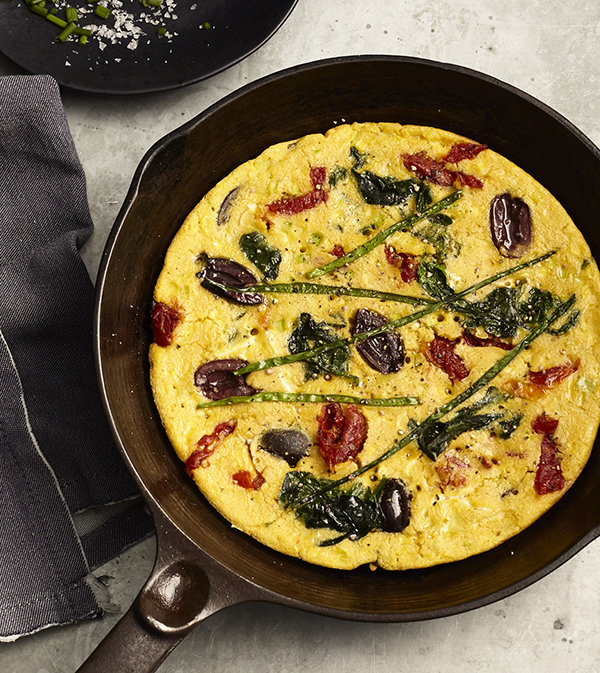A top-down food photograph showcases a well-cooked frittata in a round, brown metallic cast iron skillet. The bright yellow frittata is filled with various vegetables and garnishes, including vibrant red sun-dried tomatoes, possible olives, long green asparagus, and specks of chives and chili. The frittata's edges are slightly puckered, suggesting it might be a touch overcooked. This delightful dish rests on a white stone countertop, accompanied by a pale gray towel on the left and a black plate with chives and salt scattered on it, positioned towards the top of the image. The scene is beautifully composed, highlighting the textures and colors of the frittata against the minimalistic background.